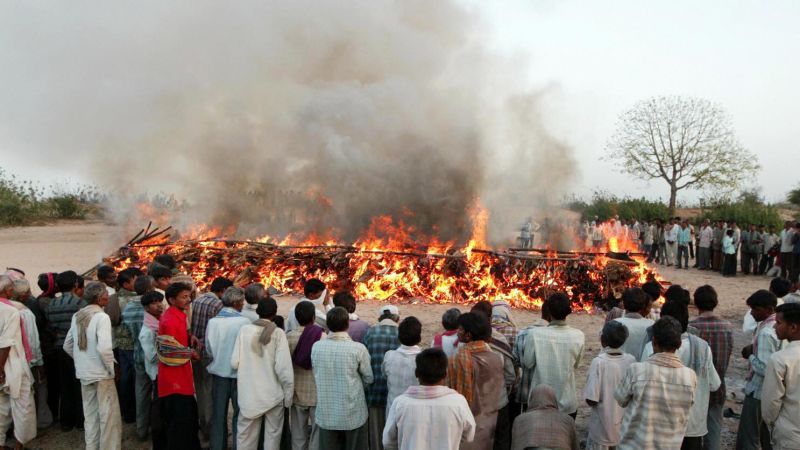This outdoor photograph captures a communal gathering centered around a large, controlled fire that seems to be part of some ceremonial or ritualistic event. The sky, partly obscured by light clouds and smoke from the bonfire, hangs over a sandy, light tan ground where around 100 men, mostly of Black or Middle Eastern descent, stand in a circle at a safe distance, observing the flames. The men predominantly wear light-colored clothes—mainly whites and grays, with some light blues—while their dark hair, styled up, adds contrast. Trees with sparse or no leaves flank the scene on both the left and right sides. The massive fire, roughly the size of four passenger cars, sends a thick cloud of smoke into the sky, contributing to the overcast appearance of the day. The participants appear calm and attentive as they watch the fire burn, accentuating the ritualistic and intentional nature of the event.